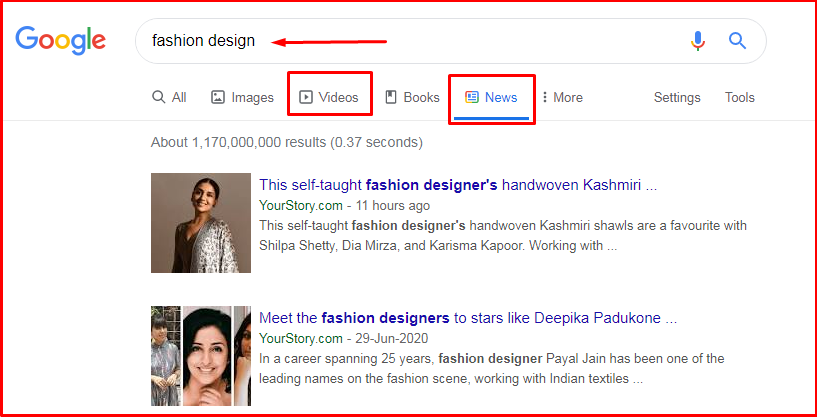In this image, set against a white background, we are viewing a screenshot of a Google search results page. In the upper left corner, the Google logo is prominently displayed, spelled out as "G-O-O-G-L-E." To the right of the logo is a search bar, within which the query "fashion design" is typed in dark gray text. An edited red arrow is pointing to the search term "fashion design." The entire screenshot is enclosed within a red border.

Below the search bar, a horizontal menu displays several categories from left to right: "All," "Images," "Videos" (which is highlighted in red), "Books," "News" (with a blue underline indicating it is the current selection, also bordered in red), "More," "Settings," and "Tools."

Further down, the first search result is visible. The title, written in blue text, reads, "This self-taught fashion designer's hand-woven Kashmiri." To the left of this title, there is an image of an attractive woman with dark hair, wearing an animal print shirt.